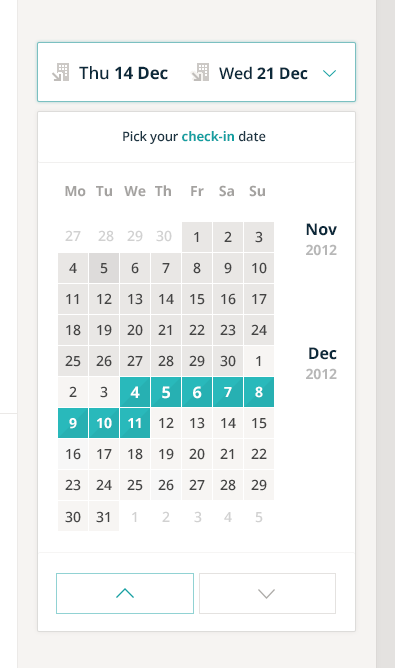A screenshot from a rental booking notification website taken in November 2012 displays an interface prompting users to select their check-in date. The visible date range for selection spans from Thursday, December 14th to Wednesday, December 21st, 2012. The calendar view shows the months of November and December 2012, with the current date marked as November 5th, 2012, distinguished by a different color. Notably, all dates in November are grayed out, indicating their unavailability for booking. The user seems to have selected the dates from Wednesday, December 4th to Wednesday, December 11th, which are highlighted in green, signifying their availability.